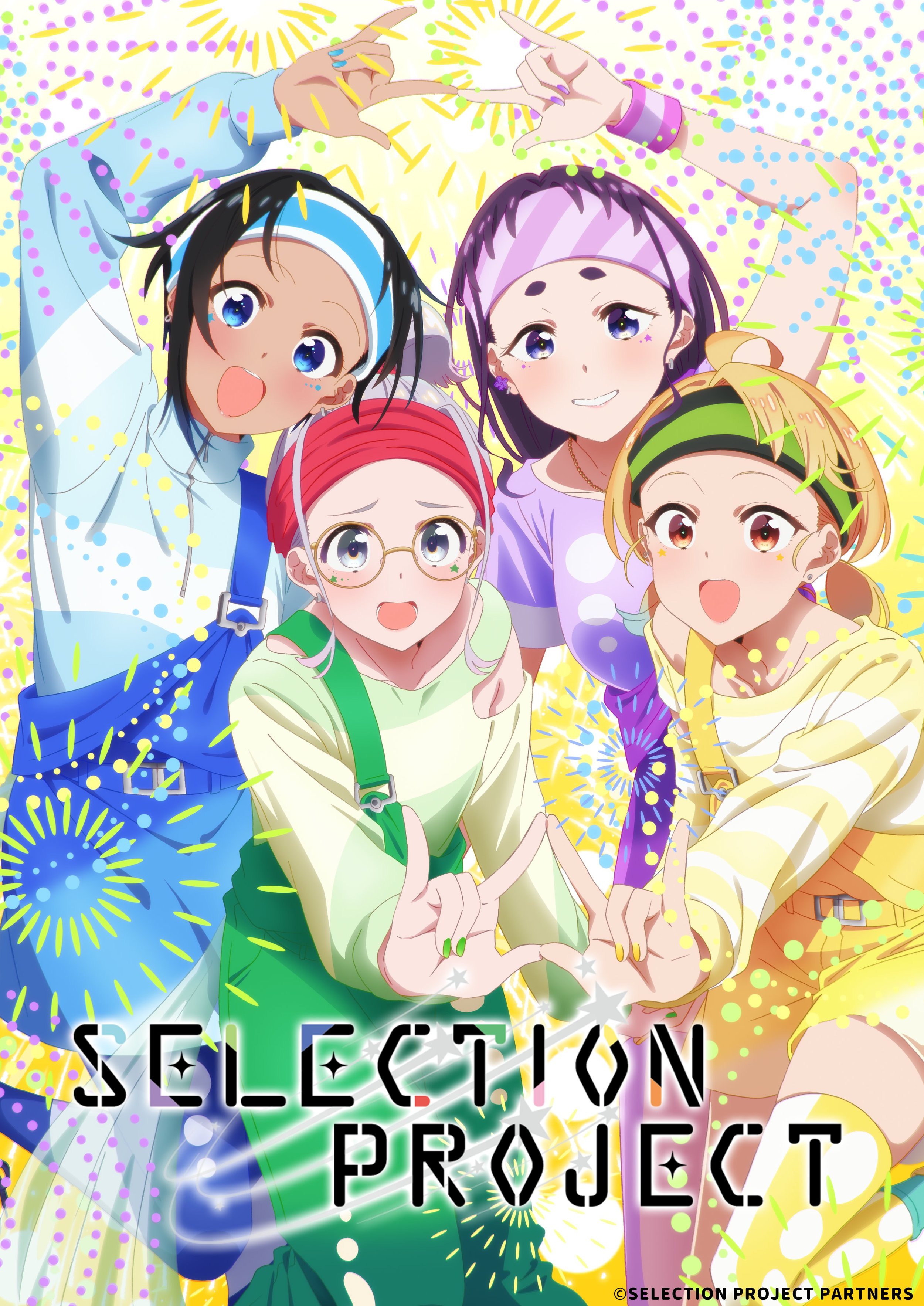The image is a vibrant, anime-style illustration titled "Selection Project," prominently displayed in black letters at the bottom, with "Selection Project Partners" written beneath. The background is a lively yellow adorned with multicolored starburst designs and dots. There are four distinct girls, each striking dynamic poses with their arms raised or extended. 

- On the far left stands a girl clad in various shades of blue, from her shirt and headband to her shoulder bag. She has blue eyes and blue-painted fingernails that complement her outfit.
- Next to her is a girl in purple attire. She has violet eyes, a purple headband, bracelet, and fingernails, creating a cohesive look.
- In front, a girl with glasses and gray eyes is adorned in green coveralls and a red headband, extending her right hand forward. Her fingernails are painted green.
- To her right, another girl is dressed in yellow overalls, wearing a green and black headband. She has brown eyes and yellow-painted fingernails.

The characters' large, expressive eyes, characteristic of anime, add emotion to the scene, which is filled with vibrant colors and energy, making it feel like a promotional poster for a show or game.